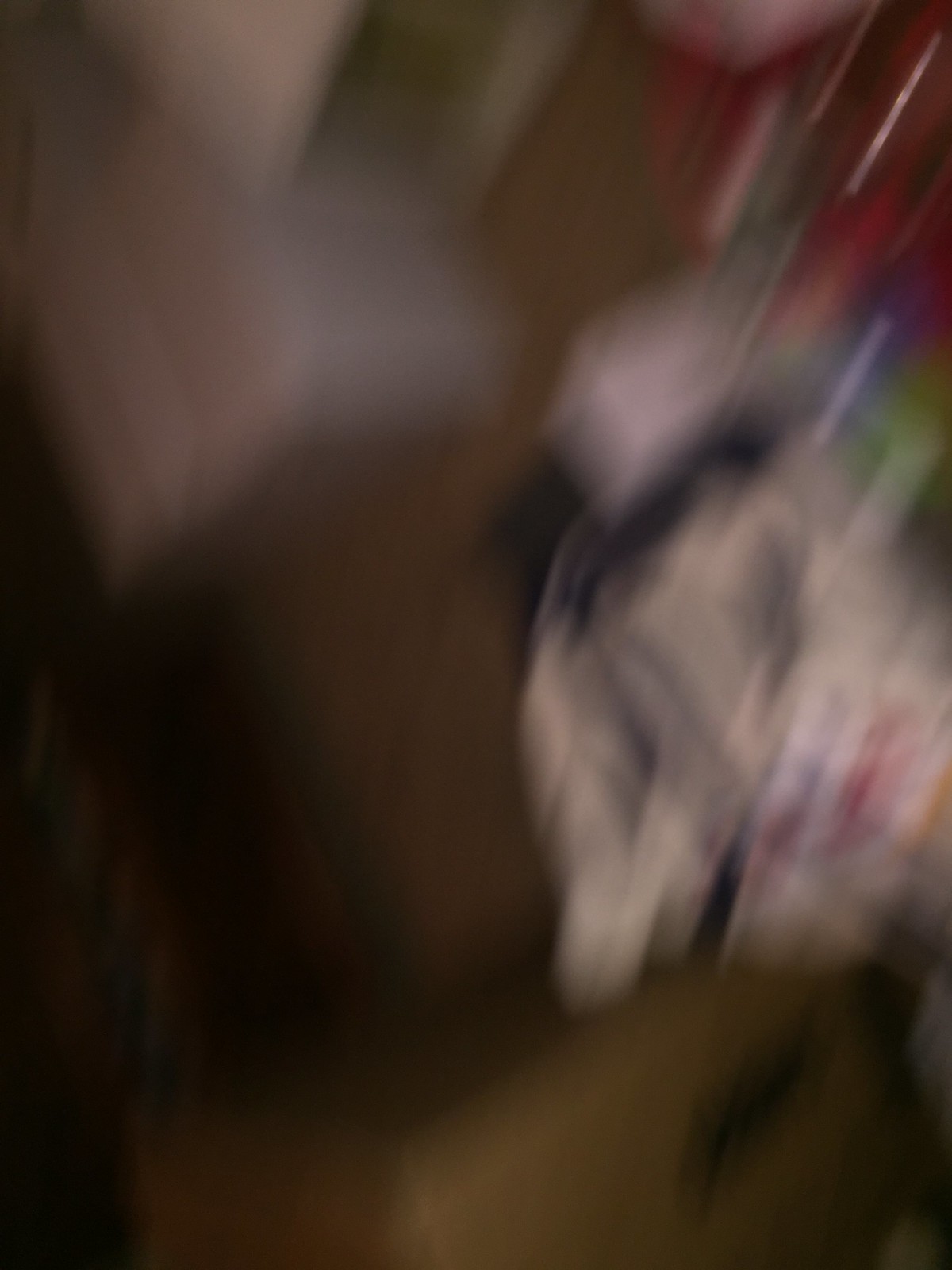The image is extremely blurry, making it challenging to discern specific details. In the center, there appears to be a brown object, possibly a chair with an armrest, flanked by another indistinct brown square. Toward the center-right, there's the hazy outline of what might be a face, discernible by a protruding nose, potential hair, and possibly red lips. Additional colors such as red, blue, and green are scattered throughout, though their exact nature is obscured by the blurriness. The rightmost part of the image features a large white area that could be piles of something, with the background showing some red and white hues and a darker left corner. There are no clearly identifiable writings, people, animals, signs, plants, flowers, or trees in this very indistinct photograph.